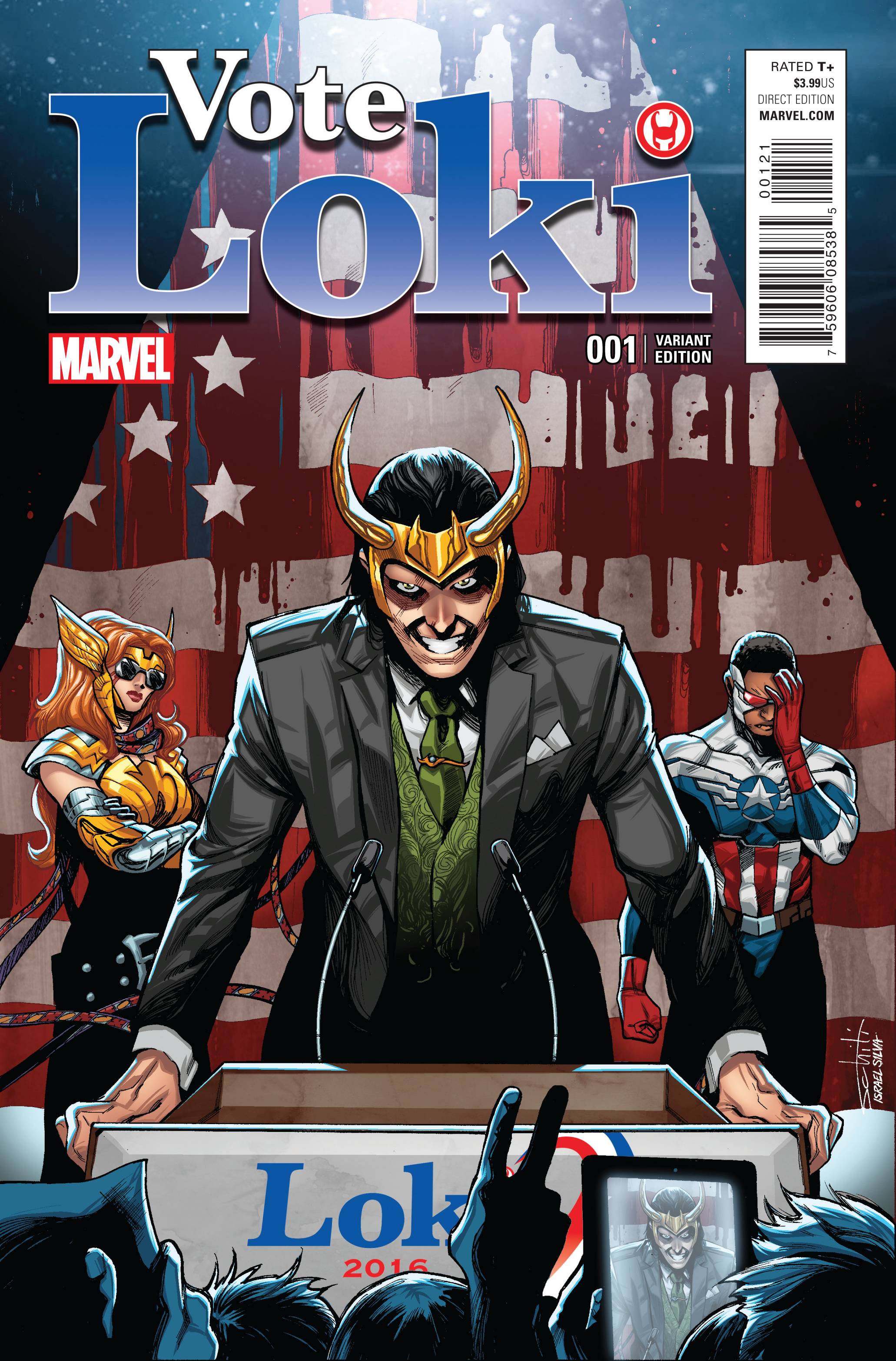The cover of the comic book "Vote Loki" by Marvel depicts Loki standing at a podium labeled "Loki 2016." At the top of the image, the title "Vote Loki" is prominently displayed in white and blue lettering. Loki is centered on the cover, wearing a black suit with a green waistcoat, a green tie, and a golden crown with large, curved horns. His long black hair falls behind him, and he sports a grin as he grips the sides of the podium, which has two microphones.

In the background, a triangular section of the American flag appears to have blood dripping from the red stripes. To Loki's left stands a woman with orange hair, clad in a gold and silver metallic outfit with eagle ears. To his right is a man wearing a Captain America suit, characterized by its red, white, and blue patriotic colors, and red sunglasses covering his eyes.

In the foreground, partially visible heads and silhouettes of the audience are seen, some holding signs, making peace signs, and recording Loki on their phone screens. The cover is marked as issue 001, a Variant Edition, with a rating of T+ for teens and up, priced at $3.99, and includes the Marvel.com logo along with a UPC code.